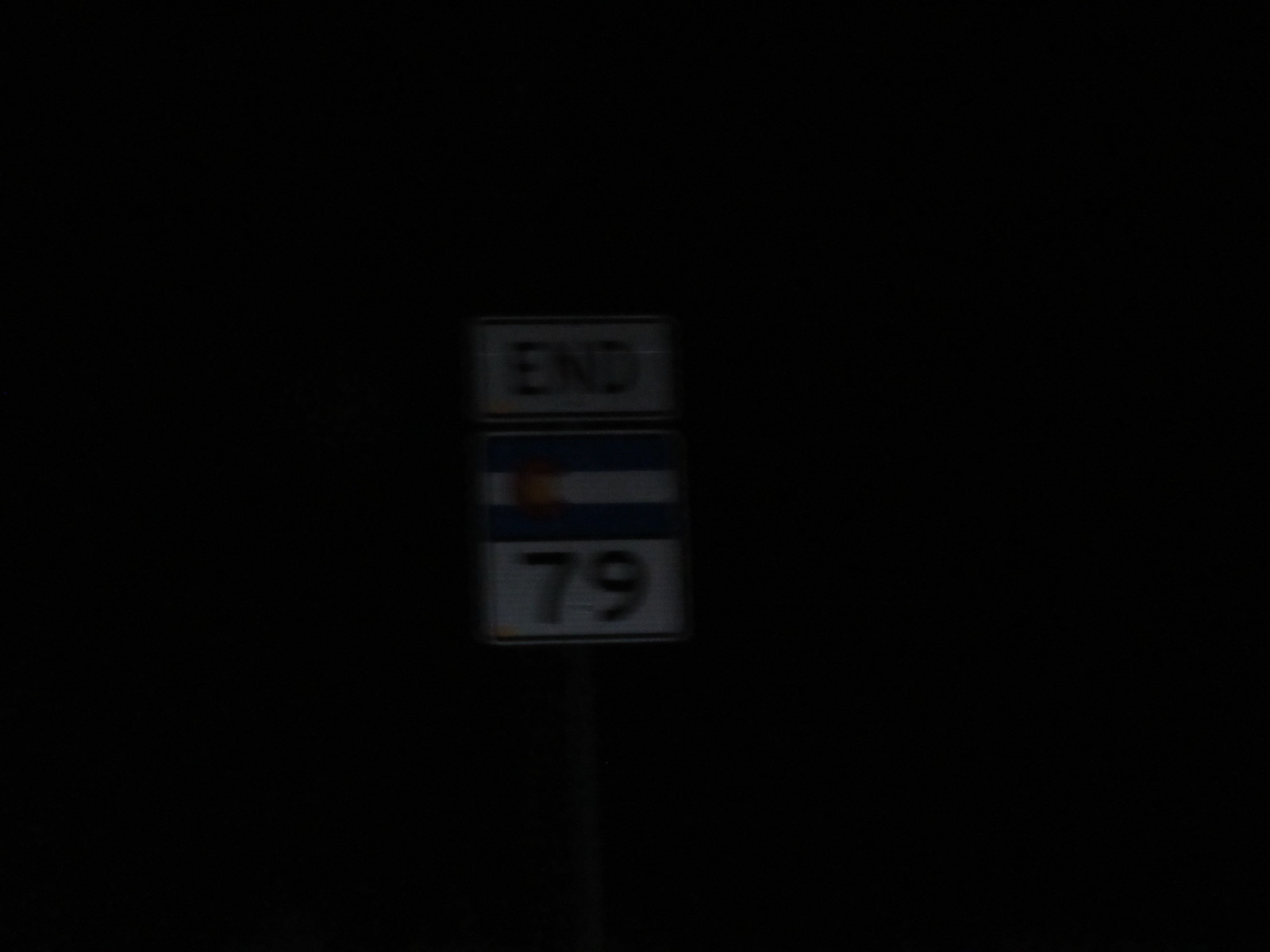In this extremely dark and somewhat blurry night-time photo, the central focus is a small street sign composed of three sections. The top section is a white rectangular background with the word "END" in black text. Below it lies a pattern of cobalt blue and white rectangles, reminiscent of the Colorado state flag, with a red medallion-like logo on the left. The bottom section displays the large number "79" in black against a white backdrop. The sign, mounted on a thin dark pole, seems to be a type of road or street sign not commonly found in the United States. The surrounding environment is pitch black, devoid of any light sources, making the sign the sole visible element in the photo.